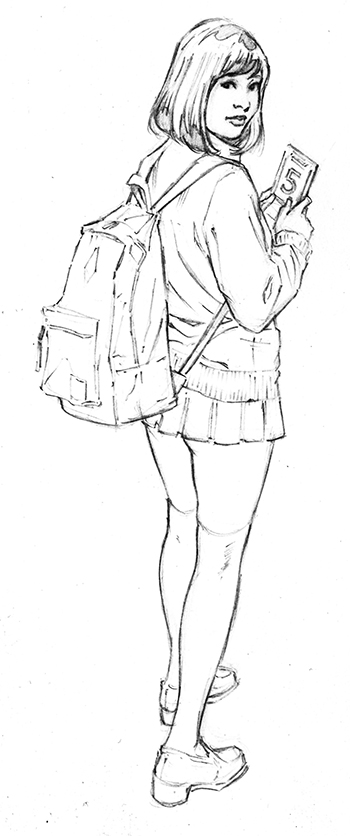This is a detailed black-and-white pencil sketch of a young woman, possibly aged from her teens to mid-twenties. She has a medium-length bob haircut with bangs, her hair falling just below her chin. The woman is seen from behind but is turning her head over her right shoulder, gazing back at the viewer. She is adorned in a jacket and a very short pleated skirt, so short that it reveals the start of her buttocks. Her outfit is completed with knee-high stockings and loafers with a slight heel. She carries a backpack and holds a square card or smartphone-like device displaying the number "5." The background is plain and white, emphasizing the central figure. The drawing conveys a retro vibe, perhaps reminiscent of the 1960s.